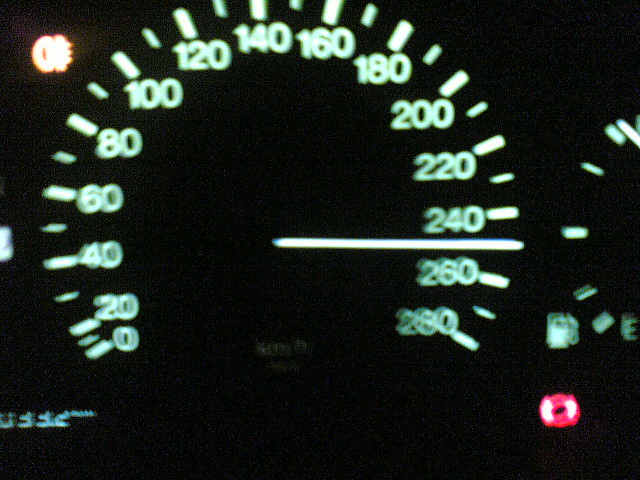The image displays an intricate speedometer. Starting from the bottom left and curving in a circular arc to the bottom right, the numbers begin at 0 and increase by increments of 20, reaching up to 280. Each number is accompanied by small dashes, with additional dashes placed between each number to mark 10 mph increments. A prominent white line points towards the 250 mph mark, indicating the current speed or the position of the needle.

To the right of the speedometer, there is a smaller, half-circle gauge composed of tiny dots and dashes, with an 'E' at the bottom, possibly representing an empty fuel indicator. To the left of this gauge is an icon resembling a gas station pump, and below that is a small red circle, which could indicate a warning or alert.

Above the speedometer, on the left side, a yellow circle is visible, accompanied by an indescribable symbol. At the bottom of the screen, there are additional numbers, reading '0332' or something similar, hinting at an odometer or trip meter reading. The detailed dashboard provides a comprehensive look at various indicators and measurements for the vehicle.